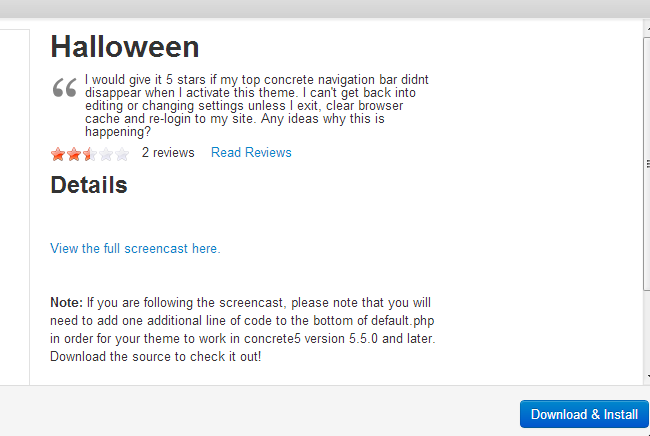**Caption:**

A detailed screenshot of various user reviews for a particular application, likely a theme or plugin for a website management tool such as Concrete5. 

The first review, prominently titled "Halloween" in large letters, highlights a user's frustration. The user mentions they would rate the app five stars if it weren't for an issue where the top navigation bar disappears upon activating the theme. This issue forces the user to exit, clear the browser cache, and re-login to make any edits or change settings. The review is rated two and a half red stars and includes two other reviews alongside it. 

To the side of the reviews, there's a prompt encouraging users to "Read Reviews." Below that, a clickable blue link says "View the full screencast here," with a note emphasizing the need to add an additional line of code at the bottom of the default PHP for compatibility with Concrete5 version 5.50 and later versions. Finally, a call-to-action button at the bottom reads "Download and Install," allowing users to easily access the source and make appropriate modifications.